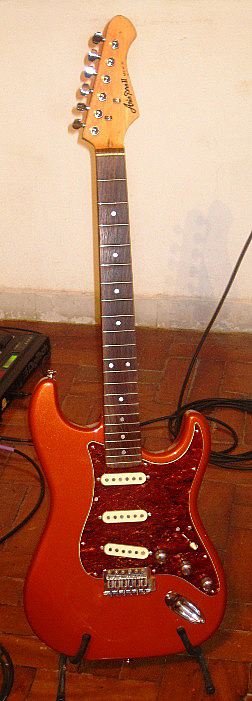The image showcases a red electric guitar resting upright on a black stand. The guitar, featuring a sparkly red and orange-red stone-like finish, appears to be a high-end model similar to a Gibson Les Paul. The body of the guitar displays a mix of light and darker shades of red, with a brown neck leading up to a headstock that has silver metal tuners. In the background, a wooden floor with a brick-like terracotta tile design and a white wall can be seen. Several cables and wires are scattered around, with a coiled cord indicating the guitar is not currently plugged in. Additionally, a black amplifier with a small green screen is visible to the left, while the base of the wall features a poorly painted dado rail.